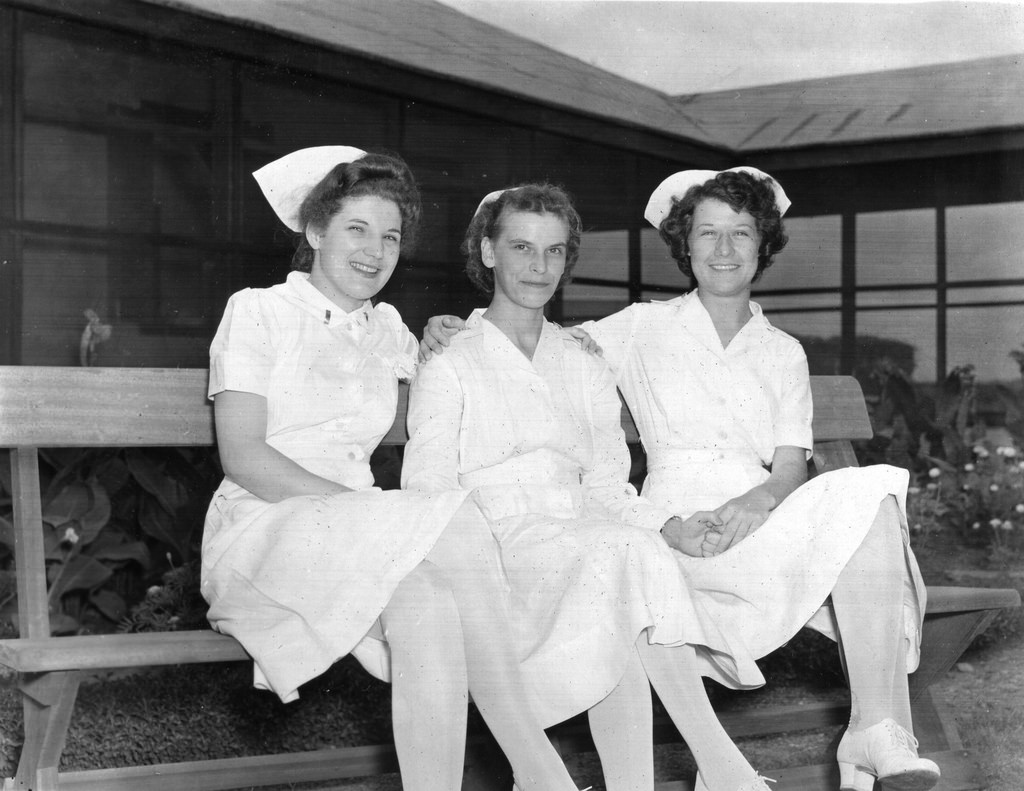In this black-and-white photograph, three female nurses are seated closely together on a simple wooden bench, positioned outdoors in front of a small building characterized by numerous windows. The setting also features a small flower garden. The nurses are dressed in traditional white uniforms: knee-length dresses, white stockings, and lace-up white shoes with modest heels. Each woman wears a white nursing cap pinned into her brunette hair, signifying their profession and era. The nurses appear to be close friends, as evidenced by their affectionate poses—arms draped around each other and hands gently clasped. Their expressions convey camaraderie; two nurses smile widely, while the one in the center sports a subtler, half-smile. The bench, described as basic with a single rail at the top and a single board at the bottom, adds an element of simplicity to this evocative and nostalgic scene, likely dated to an earlier time given their vintage attire.